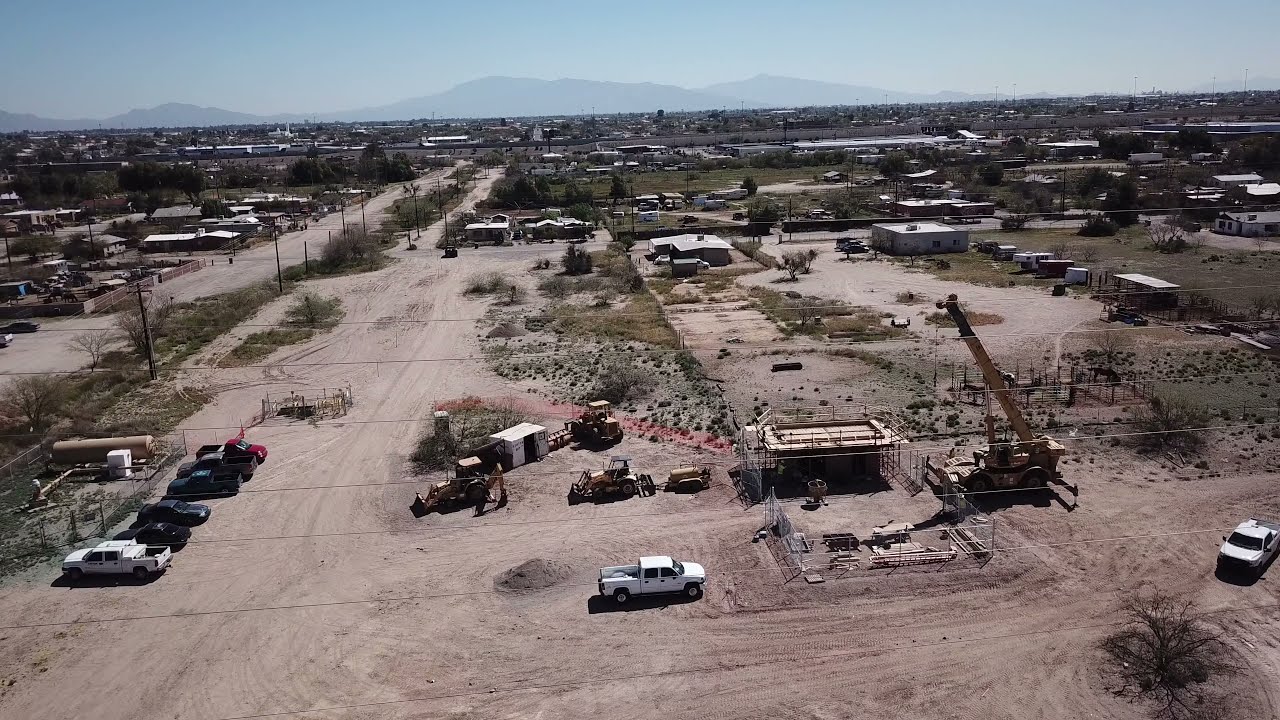This photograph showcases a valley in a desert area, captured from a high vantage point, offering a broad and detailed view of the landscape. In the foreground, there are several sandy, empty lots where various construction activities are evident. A tractor is visible in one lot, while a tall crane with its arm fully extended dominates another. The scene is populated with numerous yellow construction vehicles and pickups, signaling an active construction site. 

A dirt road runs alongside these lots, flanked by telephone poles and sparse vegetation, including some trees and patches of grass. As the eye moves further into the mid-ground, the landscape transitions to a more developed area with multiple buildings, including single-story homes and possibly mobile homes, all blending into the sandy environment. 

Far into the distance, a town comes into view, nestled at the base of three prominent mountain peaks. The sky above is clear and blue, with the sun shining brightly, flooding the scene with natural light. Notably, there are no people present in the image, emphasizing the stillness and the ongoing construction activities in this expansive desert valley.